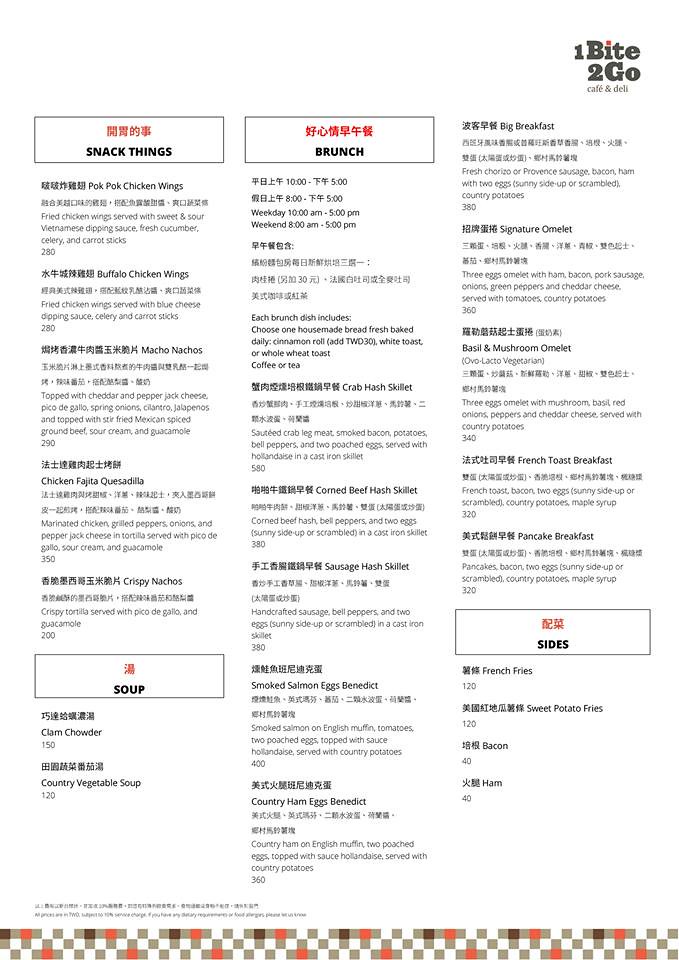The scanned image depicts a white page from a Chinese food menu. In the upper right corner, the title "One Bite, Two Go Cafe and Deli" is prominently displayed, with the words "One" and "Two" represented numerically as "1" and "2" respectively. 

On the top left, the section titled "Snack Things" is written in bold black font. This section lists a variety of snack items including:
- Pock Pock Chicken Wings
- Buffalo Chicken Wings
- Macho Nachos
- Chicken Fajita Quesadilla
- Crispy Nachos

Beneath this is another bold-font section labeled "Soup," offering:
- Clam Chowder
- Country Vegetable Soup

In the middle of the menu, a bold-font heading reads "Brunch," underneath which a diverse array of brunch options are listed:
- Crab Hash Skillet
- Corned Beef Hash Skillet
- Sausage Hash Skillet
- Smoked Salmon Eggs Benedict
- Country Ham Eggs Benedict
- Big Breakfast
- Signature Omelet
- Basil and Mushroom Omelet
- French Toast Breakfast
- Pancake Breakfast

Each section is clearly defined, making it easy to navigate through the varied offerings of snacks, soups, and brunch items.